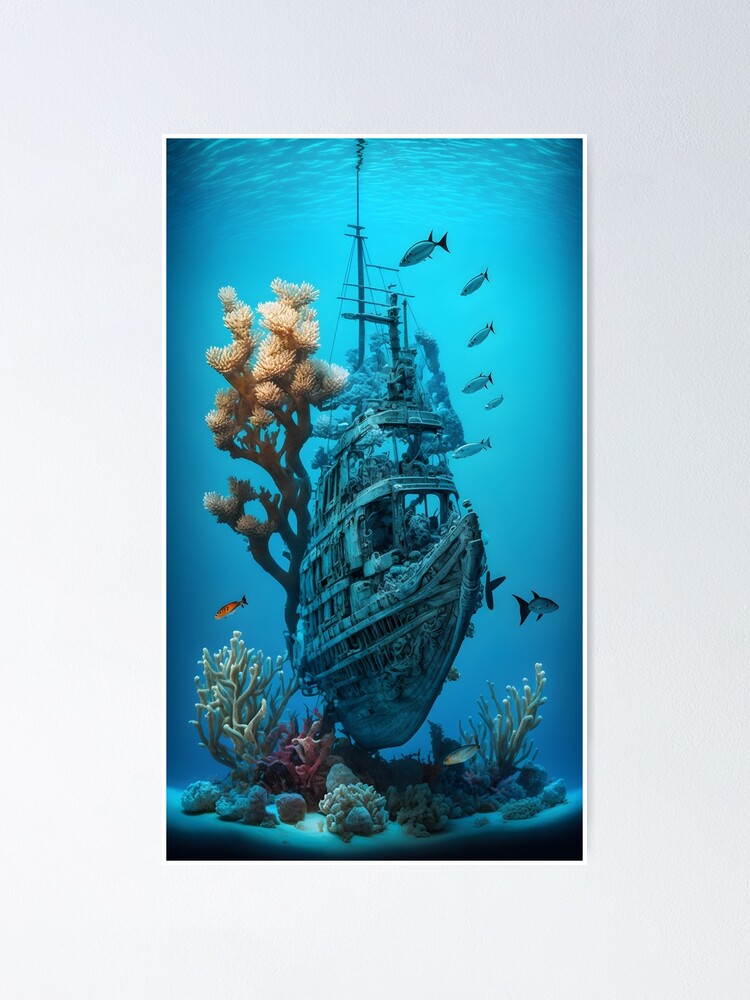The image is a framed painting of a sunken wooden ship, displayed on a wall with a thick, light gray, almost white border. The ship, depicted in a deep, bright blue ocean, stands upright, partially deteriorated with numerous missing planks and a tattered flag. Coral and barnacles encrust its hull, with a particularly large piece of coral growing towards the top of the ship. Various fish, predominantly to the right of the vessel, swim in and around it, with one distinct red fish visible to the left. The blue-tinted water adds depth to the scene, completing the mesmerizing underwater tableau.